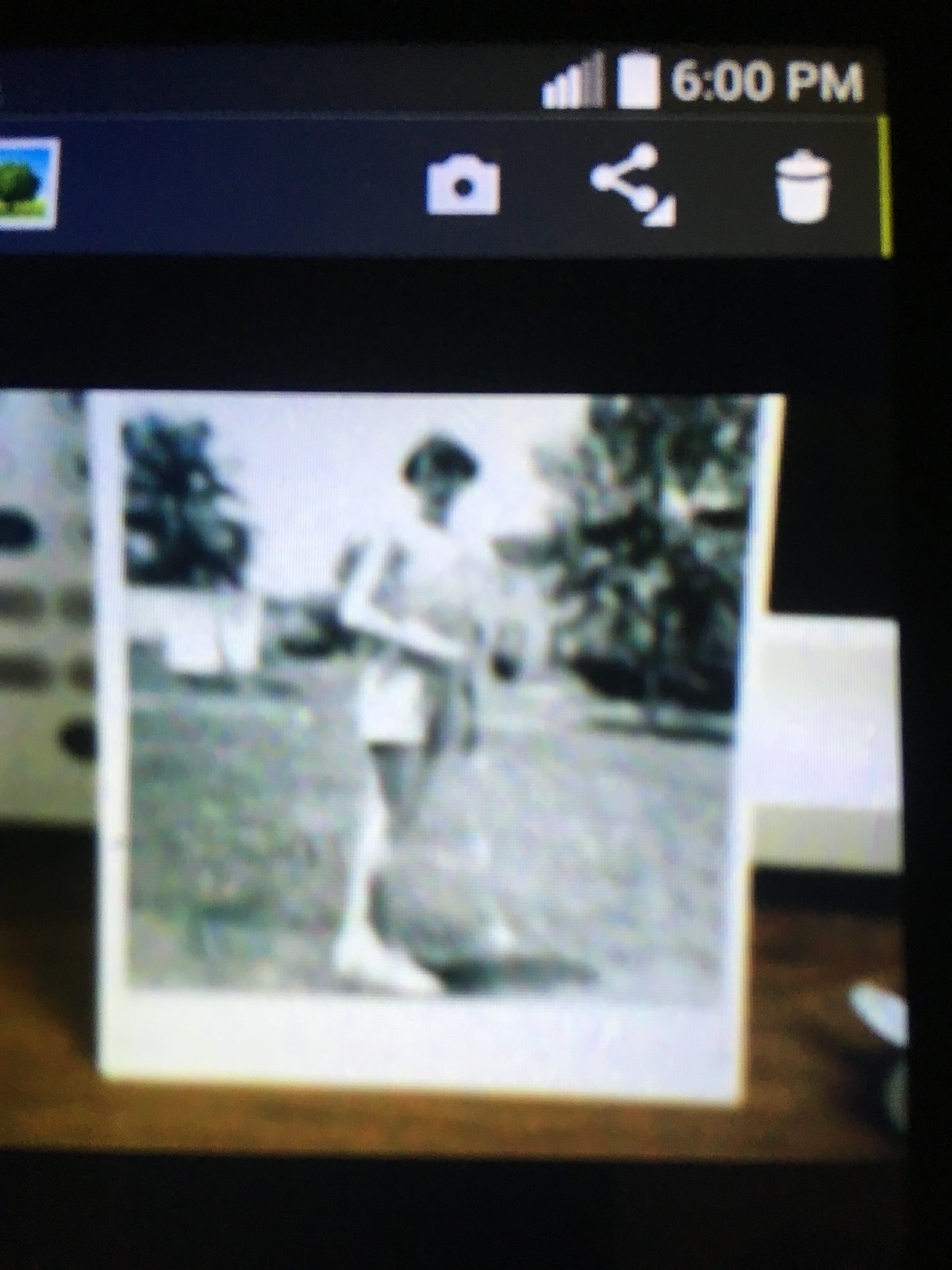The image depicts a somewhat blurry close-up of a tablet screen, possibly an iPad, displaying a black-and-white Polaroid photograph. The tablet screen indicates the time as 6:00 p.m., and shows a 3-bar Wi-Fi signal along with a full battery charge in the corner. On the top left of the screen, icons for trash, photo, camera, share, and download are visible. The Polaroid photograph itself captures a sunny day, showing a woman standing outside in a yard with short grass and trees in the distance. She is dressed in a jumper, shorts, and tennis shoes, looking directly at the camera. The Polaroid appears to be resting on a brown wooden surface, possibly leaning against a wall or a basket, adding depth to the scene.